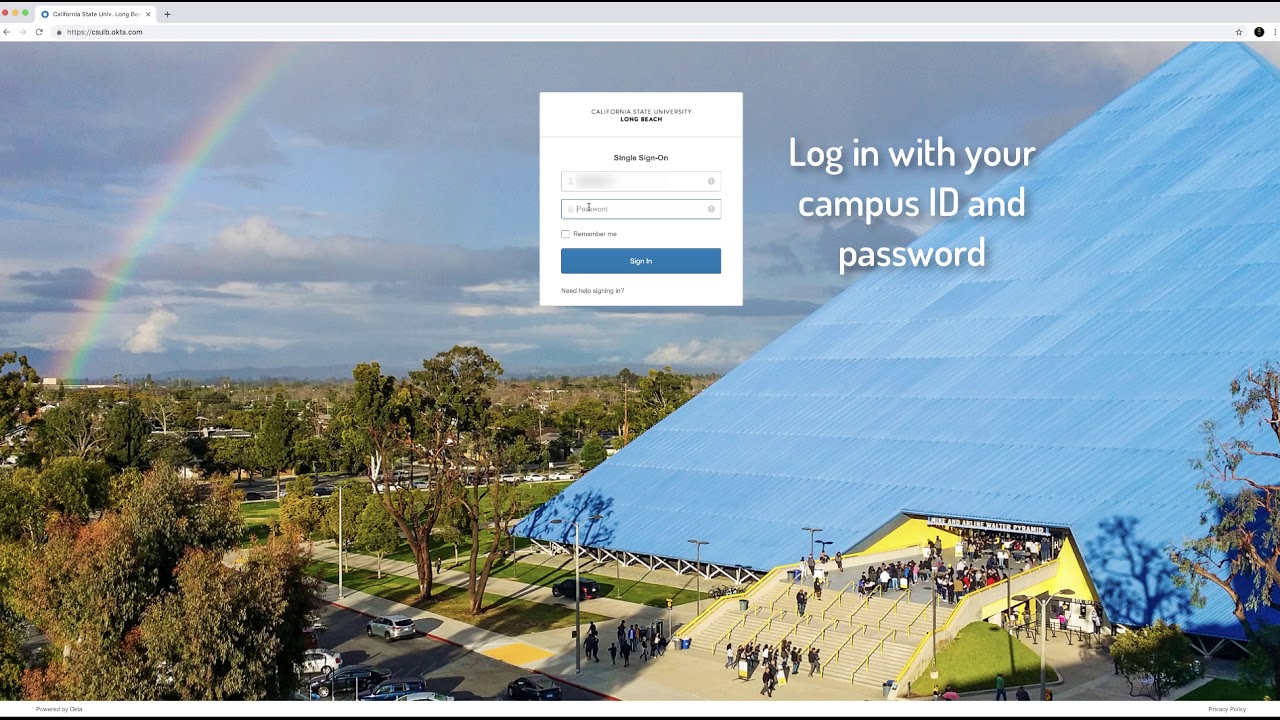The screen displays a web page open on a browser, specifically for California State University, Long Beach. The URL reads "csulb.okta.com". The focal point of the image is a rectangular photograph that partially shows the pyramid sports complex, capturing just one side of the structure extending upwards but not the entire pyramid itself. 

The interface is inviting the user to log in with their campus ID and password. There is a prominent white rectangle vertically aligned, with the text "California State University, Long Beach" at the top. Below this is a grey horizontal line, followed by the text "Single Sign-On".

The login area consists of two primary fields; the first is the 'Name' field, which is currently greyed out and obscured, and the second is the 'Password' field, surrounded by a blue outline indicating it is active, though no text has been entered yet. The cursor is positioned within this password field. Underneath these fields, there is an unchecked "Remember me" checkbox. Further down, there is a teel blue button, matching the width of the login fields, with white text instructing "Login".

At the bottom, the web page provides a "Need help signing in?" link for additional support.